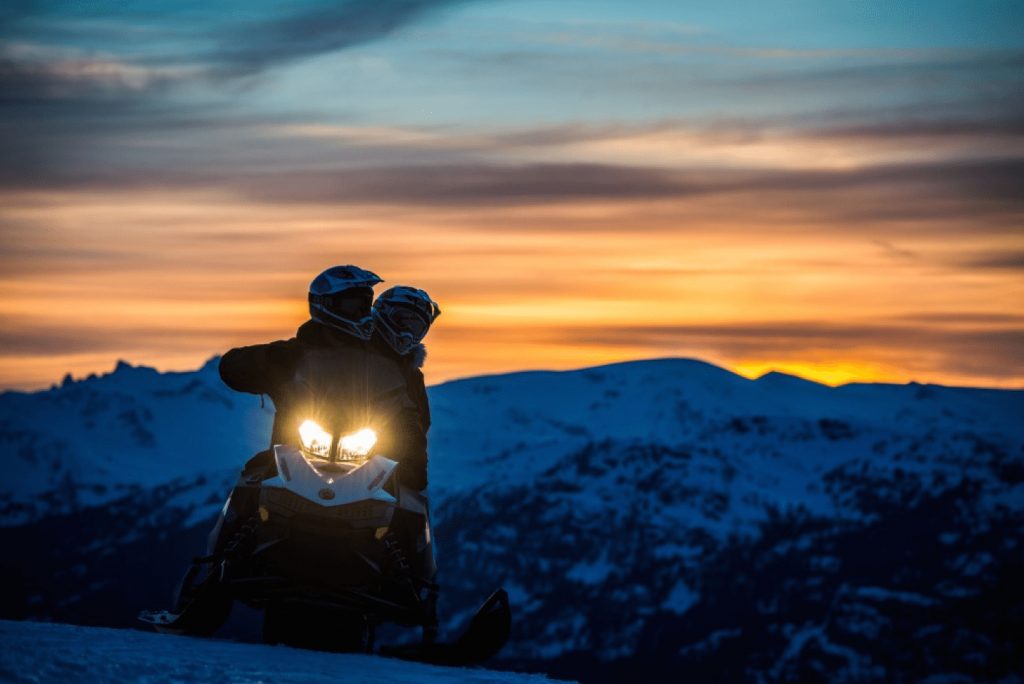In this striking painting, a couple is captured in an intimate embrace while sitting on a snowmobile atop a snowy hill or mountain, bathed in the enchanting light of a setting sun. The couple, both wearing helmets and black coats, are silhouetted against the vibrant backdrop, their features obscured by shadows. The snowmobile, adorned in black and white, has its headlights on, casting a dim glow that adds to the romantic ambiance. In the distance, the landscape is framed by majestic, snow-capped mountains that transition from dark, rocky peaks to serene, blue slopes. Above, the sky is a mesmerizing tapestry of vibrant colors—deep blues, grays, pinks, yellows, and oranges—that blend together to paint a breathtaking sunset. The ethereal light from the sky not only illuminates the snow, giving it a bluish hue, but also casts a soft, navy blue tint over the entire scene, encapsulating the couple in a moment of peaceful twilight.